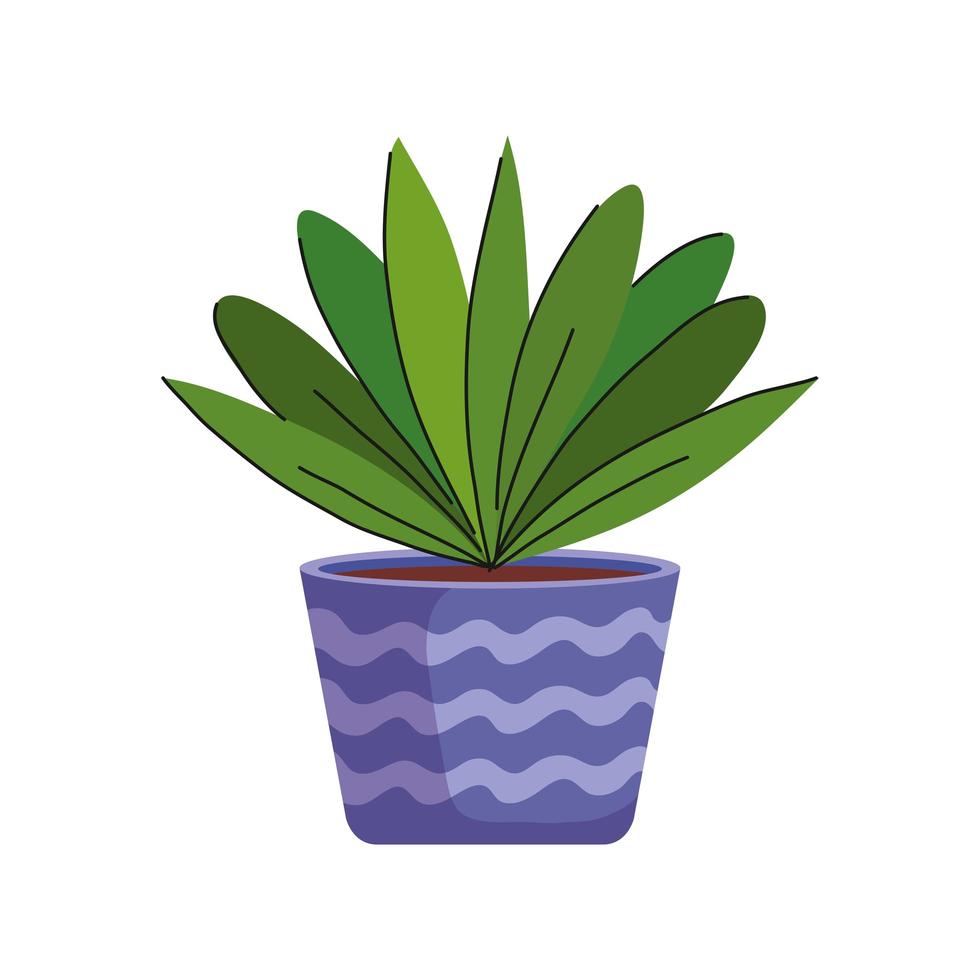The image is a cartoon drawing of a plant in a pot against a blank white background. The pot is a purplish-blue color with three lighter purple wavy stripes evenly spaced horizontally. It contains brown dirt, depicted without texture. From the pot emerges a plant with nine leaves, each resembling elephant ears and fanning out in various directions. The leaves exhibit a range of green shades, from light to dark and medium, with some featuring a central black line. The pot also has shadows adding a touch of realism to the cartoonish style of the image.